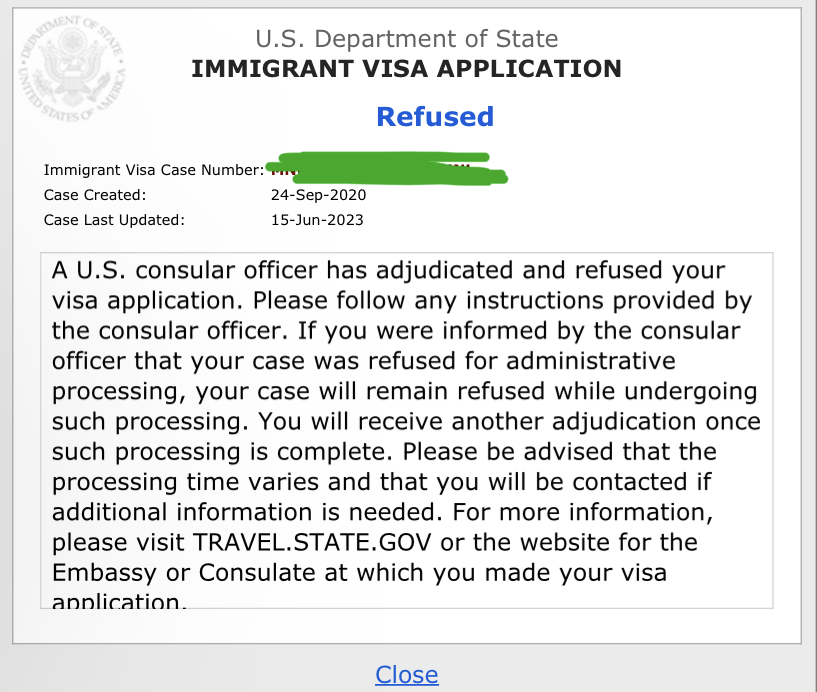The image displays a screenshot from the U.S. Department of State's immigrant visa application portal. In the top-left corner, the seal and insignia of the Department of State, United States of America, are visible. The main content of the image reveals various details about an individual's visa application.

The text states that the "Immigrant Visa Case Number" field is present, but the actual number has been obscured with green scribbles to maintain confidentiality. The case was initiated on September 24, 2020, and last updated on June 15, 2023. The status of the application is marked as "Refused."

A detailed explanation follows, indicating that a U.S. consular officer reviewed and denied the visa application. The message instructs the applicant to follow any specific directions given by the consular officer. It notes that if the refusal was for administrative processing, the case would remain in the "Refused" status until such processing is complete. The applicant will receive further communication once the processing concludes, although processing times can vary. Additional information can be sourced from the website travel.state.gov or the specific embassy or consulate where the application was made.

At the bottom of the screenshot, there is a "Close" hyperlink, which allows the applicant to exit the portal. The essence of the image is that the individual's immigrant visa application was refused, with updates and actions spanning a three-year period.